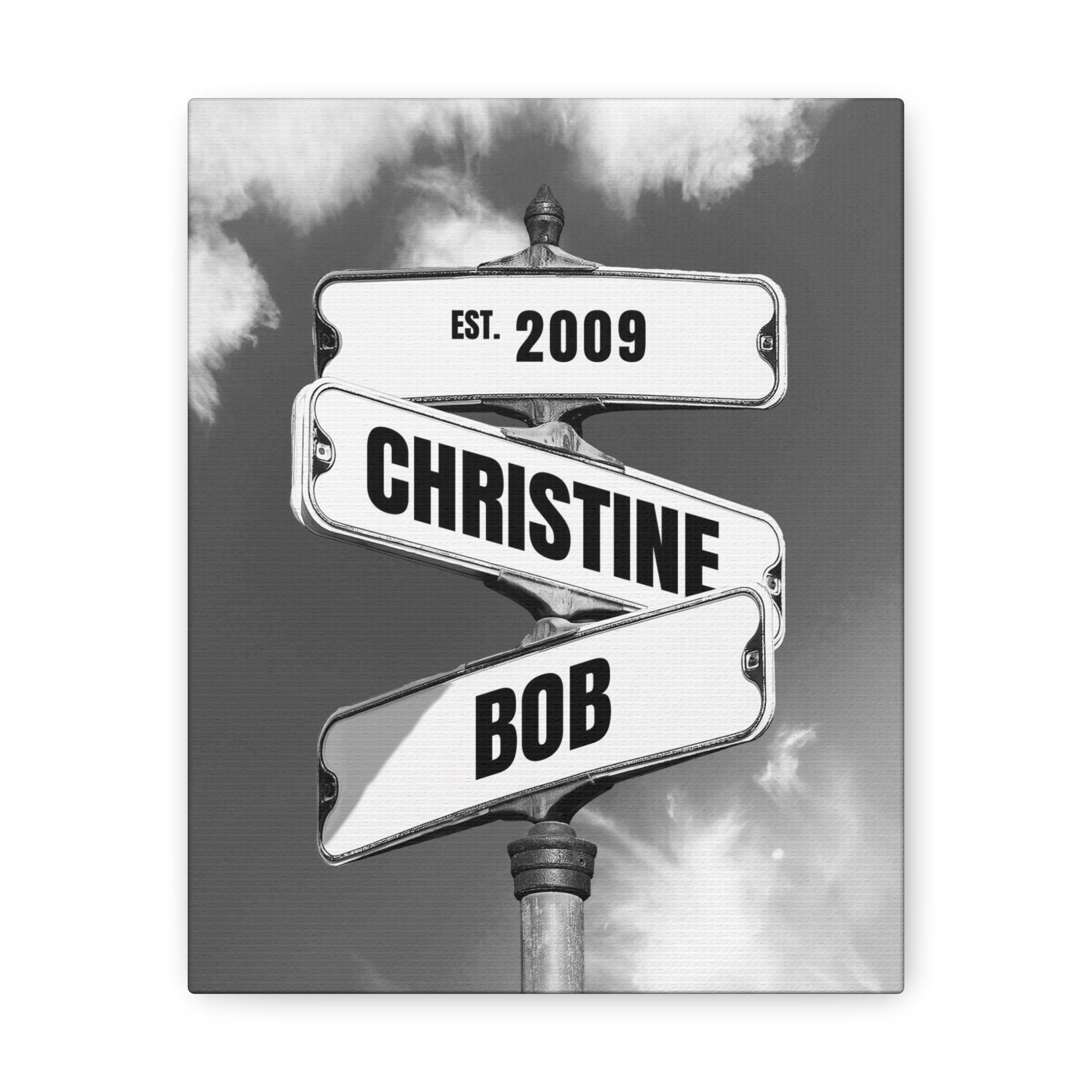This black-and-white photograph captures a vintage-style signpost featuring three distinct street signs angled in different directions. At the top of the metal pole, the highest sign reads "EST 2009" in bold black lettering. Below it, the middle sign displays the name "Christine" in equally prominent black letters, and the bottom sign, also in bold black text, says "Bob." The signpost is set against a gray sky dotted with white clouds, creating a stark contrast. The signs are white with black, bold text and metal frames, and the entire image is rendered with a drop shadow and a thin dark gray outline, giving it a polished, possibly photoshopped appearance. The focused composition emphasizes the top of the pole and the directional sings, suggesting both timelessness and personalization.